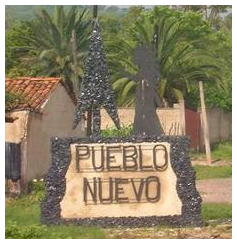This image depicts a small, iron sign with stone accents displaying "Pueblo Nuevo," seemingly situated at the entrance of a neighborhood, town, or resort. Set against a backdrop of real and possibly stylized trees, there is a mixture of tropical greenery and some foliage resembling Christmas trees. Spanish-style buildings with clay tile roofs and the warm hues of tan, orange, and brown add architectural interest to the scene. Additional details include a serene forest setting with no visible people or animals, a dirt road, green grass, and a short privacy wall or fence, suggesting a secluded and tranquil environment. The image gives a preview of this picturesque locale, characterized by its charming sign and lush surroundings.